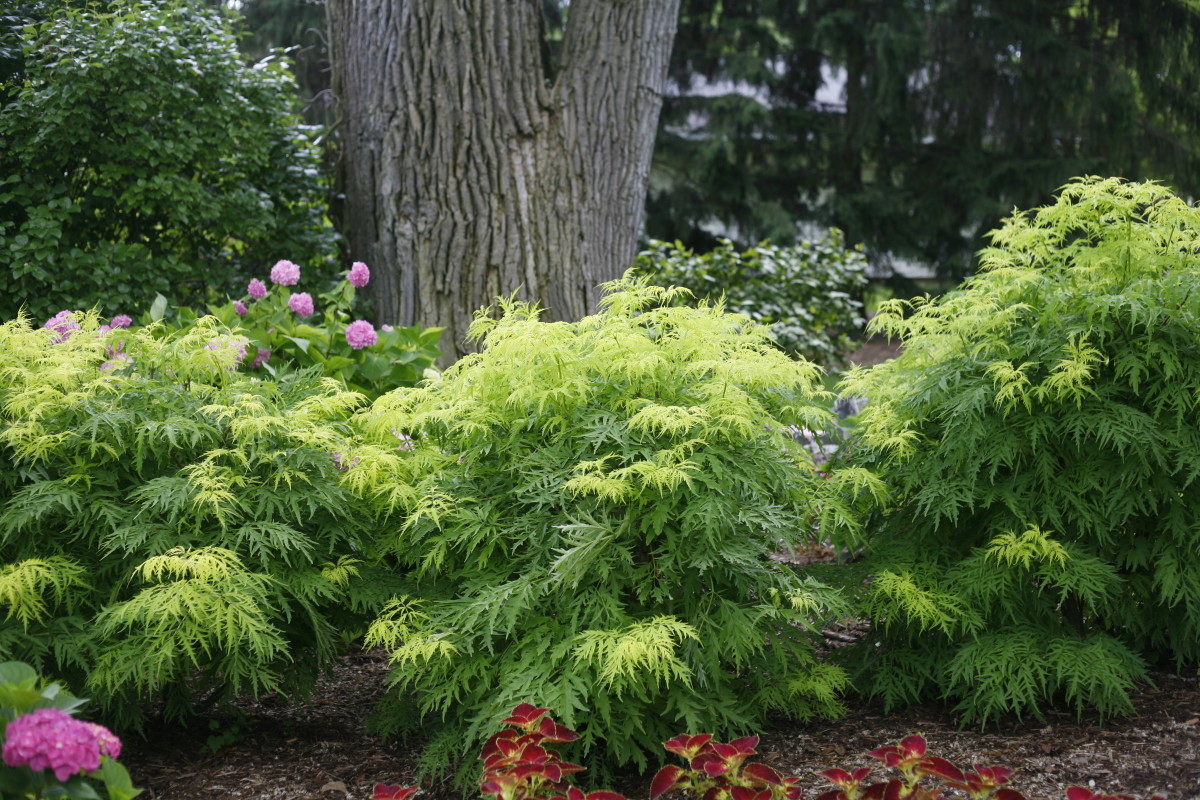This image captures a vibrant outdoor setting within a park-like garden centered around a massive and ancient tree, possibly an oak. Dominating the center, the large tree trunk branches off into a V shape, lending a sense of grandeur and age.

Surrounding the tree at ground level are a variety of lush green bushes and shrubs, characterized by their light green or yellow-green foliage. In front of these shrubs, long, spiky-leaved plants dominate the center, partially covering the trunk and adding depth to the scene. 

Vividly colorful flowers enhance the foreground; maroon and red blooms capture the eye immediately, while clusters of pink and purple flowers can be seen both to the left and scattered across the lower center and behind the greenery near the trunk. These floral elements add a dynamic contrast with their hues against the backdrop of green.

To the left of the large tree, a prominent green bush stands out, and to the right, dense trees form a leafy tapestry, with occasional glimpses of the sky signaling broad daylight. Between these natural elements, patches of ground are visible, hinting at either bare dirt or a woodchip-covered surface. The result is a richly detailed and textured portrayal of a thriving natural garden.